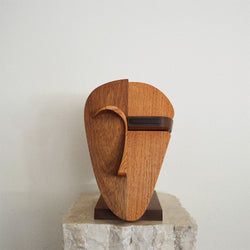This photograph features a compelling modern art sculpture, reminiscent of Picasso's style, showcasing a highly distorted and abstract wooden mask. The mask, primarily in a teardrop shape, is meticulously crafted from two distinct types of wood. The left side of the mask, made from a darker wood, features a smooth, prominent curve that suggests an eyebrow seamlessly flowing into the ridge of a nose. This side is slightly larger and elongated compared to the right. Conversely, the right side, crafted from lighter wood, is marked by a singular, thick black stripe horizontally traversing the area where an eye would typically be, giving the impression of a closed eye.

Mounted on a dark brown, possibly metal stand, the mask sits atop a unique, unfinished marble base—the top of the marble is polished, contrasting with the rough, unfinished sides. The entire composition is set against a dark cream wall, adding a striking background that highlights the sculpture's intricate details and contrasting colors.